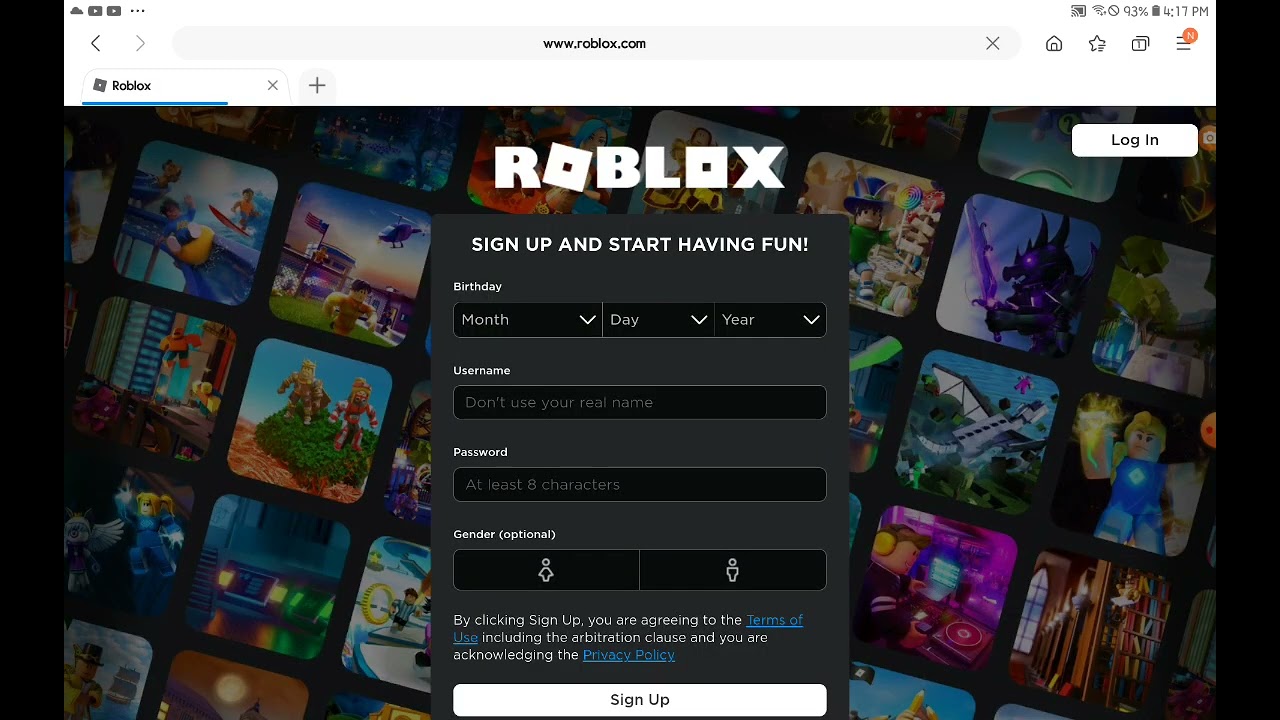The image depicts a vibrant advertisement for Roblox, presented on a web page. At the top of the page, there's a standard row of icons, followed by the URL "www.Roblox.com" displayed on a clean, white banner. 

The background of the advertisement showcases a series of frames, reminiscent of a film strip, featuring various games available on the Roblox platform, each displaying unique and colorful game graphics.

Centrally placed, the word "Roblox" takes the spotlight, stylized with the letters "R-O-B-L-O-X," where the two "O"s are designed as squares, with the first "O" slightly tilted to the right, adding a playful touch to the logo.

Beneath the logo, the ad encourages visitors to "Sign up and start having fun." The sign-up form requests the user's birthday (month, day, and year), a username, a password, and optionally, the user's gender. There is also a notice stating, "By clicking sign up, you are agreeing to terms of use, including the arbitration clause, and acknowledging the privacy policy." The phrases "terms of use" and "privacy policy" are highlighted in dark blue, making them stand out.

Additionally, there's a prominent "Sign Up" button, inviting users to complete their registration. In the upper right corner of the page, there's a small rectangular "Log In" button, providing an option for existing users to access their accounts.